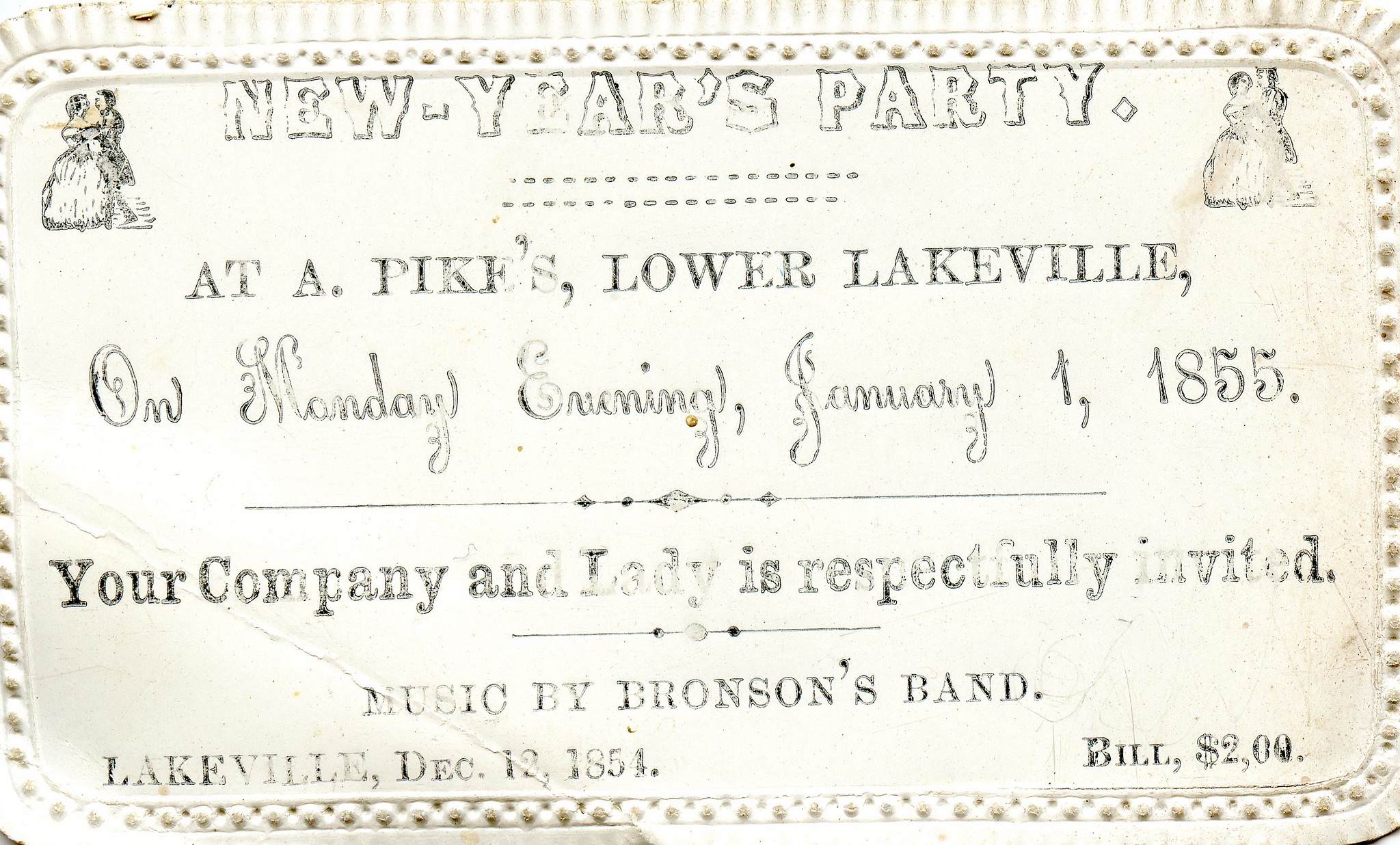This image showcases a remarkably well-preserved invitation to a New Year's Eve party held on January 1, 1855, at A. Pike's Lower Lakeville. Despite its age, the black ink text on white paper remains surprisingly legible, although some fading is evident, particularly in the stamps and illustrations. The flyer, featuring a dotted and embossed border, measures the passage of time with a single prominent crease in the bottom left corner.

The invitation's top section is adorned with illustrations of a dancing couple: the man is dressed in a tuxedo, and the woman wears a flowing white gown. The headline, "New Year's Party," appears in outline text, adding to the flyer’s charm. Below this, the main text is divided by horizontal rules and announces the details, using varying fonts, including cursive and bold lettering. It states, "At A. Pike's Lower Lakeville on Monday evening January 1st 1855. Your company and lady is respectfully invited. Music by Bronson's Band." The bottom section provides the date of issuance as "Lakeville, December 12th 1854" and lists the bill as "$2."

This invitation, with its outdated yet classic design, offers a captivating glimpse into the social events of the mid-19th century, capturing the anticipation of a splendid New Year's celebration.